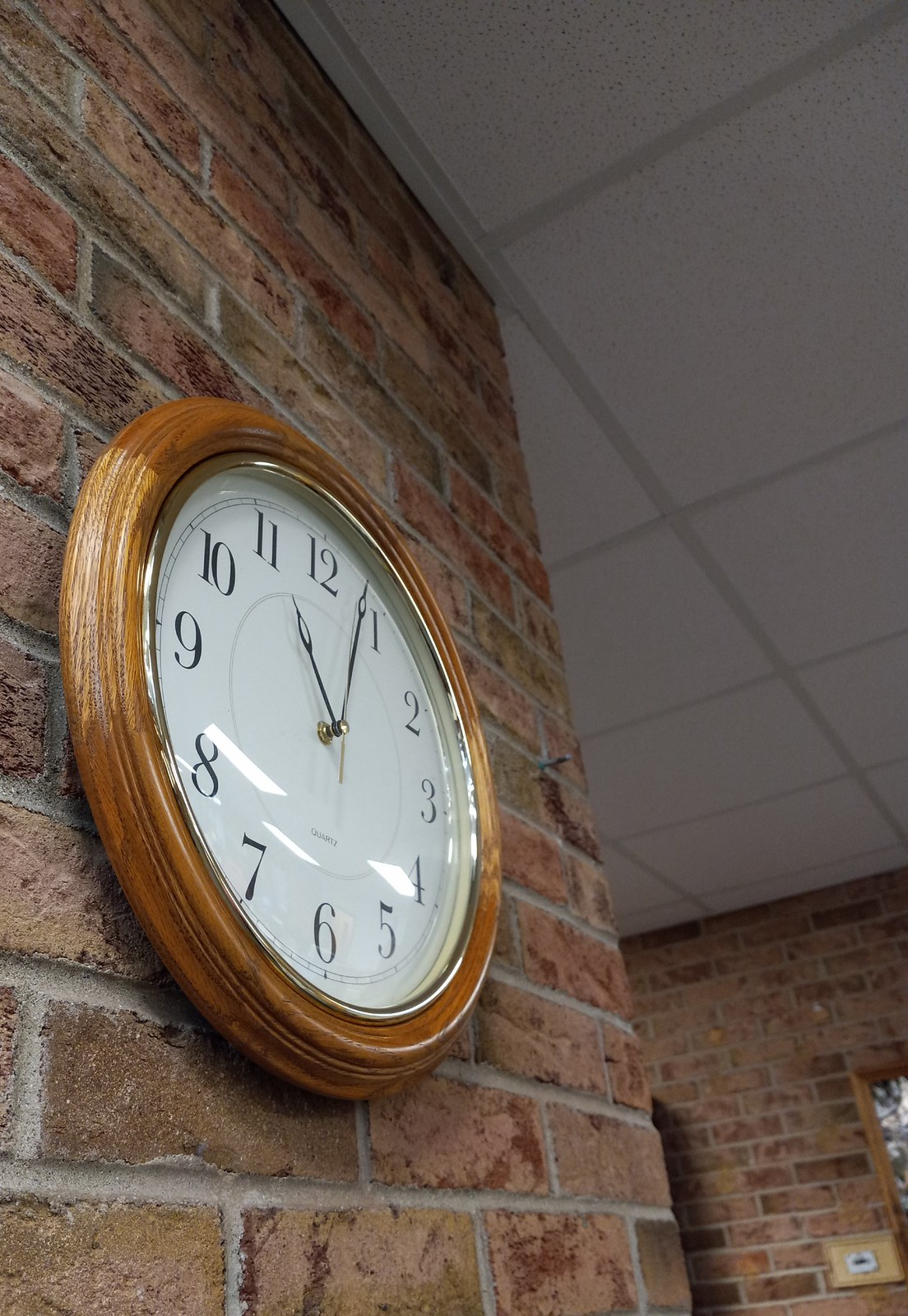This photo captures a detailed interior view featuring a wall clock mounted on a pale brick wall in what appears to be a living room. The brick wall has a subtle color palette, predominantly brown with hints of green and occasional patches of red. The gray mortar between the bricks accentuates their arrangement. 

The clock itself is a striking piece, featuring a circular exterior made of brown wood, complemented by a gold rim. The clock face is white with bold black numerals, starting at 12 at the top and continuing around the dial. The black minute and second hands are clearly visible, though the clock bears no visible brand.

In the background, the ceiling is notable for its white tiles edged with a gray border, adding a touch of refinement. Additional sections of the pale brick wall extend beyond the clock, further framing this cozy and meticulously detailed living space.